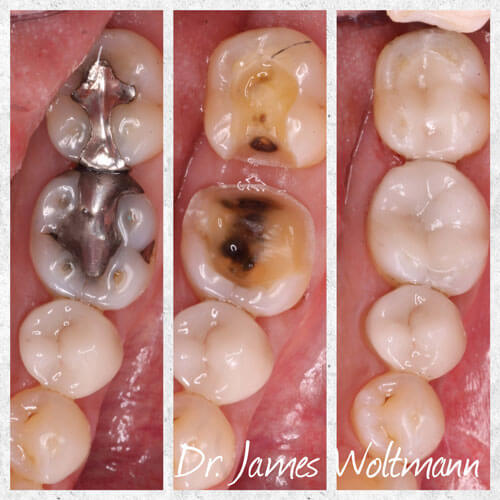This advertising image for Dr. James Noltman (spelled N-O-L-T-M-A-N) consists of three color photographs depicting the progressive dental treatment of two molars and two premolars. 

In the first photograph on the left, the teeth, situated in the back of someone's mouth, feature silver-colored amalgam fillings. The gums are visible surrounding these dental work areas. 

The middle image shows the teeth after the removal of the amalgam fillings, revealing dark discolorations and possible decay, with the areas where the fillings were appearing brown to black.

In the rightmost image, the teeth appear pristine and white, likely restored with ceramic fillings or crowns as indicated by subtle color breaks and lines. The natural-looking appearance emphasizes the transformation from silver amalgam to healthier, more aesthetically pleasing restorations.

The overall color scheme includes pinks, whites, silvers, and tans, creating a realistic and professional presentation of dental work. The text "Dr. James Noltman" is prominently displayed in white at the bottom of the photographs, attributing the dental work to the dentist.